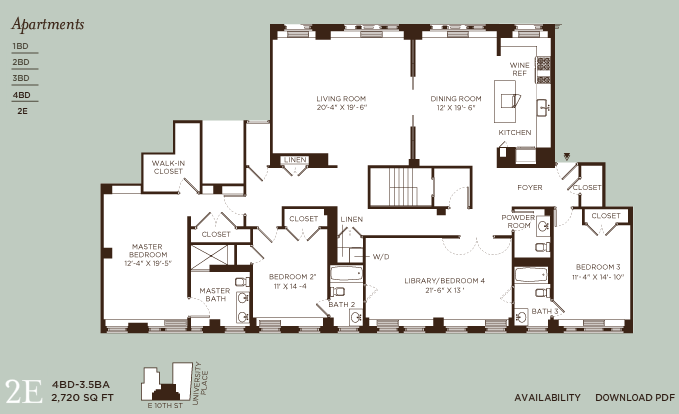This detailed diagram appears to be a floor plan for an apartment. The layout showcases various rooms and spaces in a meticulous, squared arrangement. Across the top, the rooms include a Living Room and Dining Room, adjacent to which is the Kitchen with a Wine Refrigerator. 

On the left side, the layout features a spacious Master Bedroom, complete with a Walk-In Closet, Master Bedroom Closet, and a Master Bathroom. Additionally, there is a second Closet, Bedroom, Bathroom, and two Linen closets. 

Centrally located on the floor plan is a Library and Bedroom 4. 

On the right side, you'll find Bedroom 5 (or possibly Bedroom 3), a Powder Room, two additional Closets, and a Foyer.

In the bottom left corner, there's a note specifying that the apartment includes 4 bedrooms, 3.5 bathrooms, and measures 2,720 square feet. The top-left corner indicates that the building offers various apartment configurations, including 1, 2, 3, and 4-bedroom units, and there’s notation of “2E,” although its meaning is unclear. The bottom-right corner provides information on availability and a link to download a PDF of the floor plan.